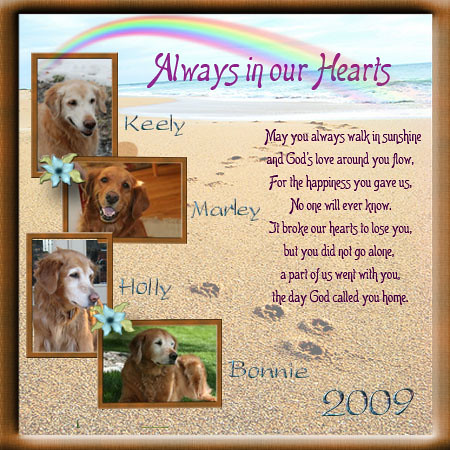The image is a framed memorial plaque, featuring four photos of golden retrievers arranged vertically on the left side, each labeled with a name: Keely at the top, followed by Marley, Holly, and Bonnie. Above the photographs is a rainbow set against a serene beach with paw prints in the sandy foreground. Prominently displayed across the top are the words "Always in Our Hearts," and to the left, in purple letters, a heartfelt tribute reads: "May you always walk in sunshine, in God's love around you, for the happiness you gave us, no one will ever know, it broke our hearts to lose you, but you did not go alone, a part of us went with you, the day God called you home." The year 2009 is inscribed in the bottom right corner, marking the date of this touching tribute.